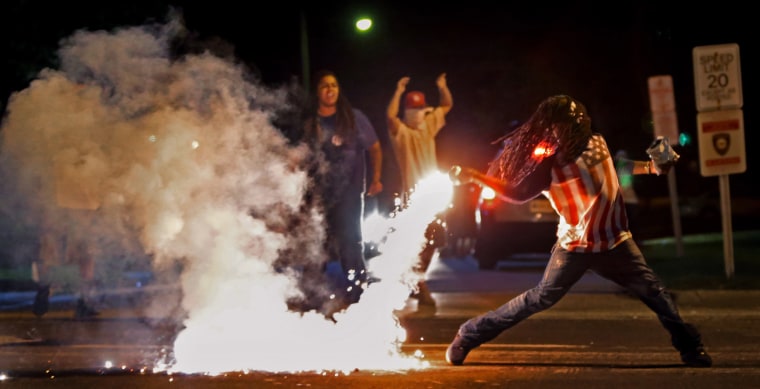In this dramatic nighttime scene set on a road, a man with long, shoulder-length dreadlocks wearing an American flag t-shirt and jeans takes center stage. He is in a dynamic pose, throwing a flaming object—likely a flare or tear gas canister—with a large blast of fire emanating from his hand, consuming a significant portion of the left side of the image. A substantial cloud of smoke trails the fiery projectile, enshrouding parts of the scene. Behind the main figure, a man in a yellow shirt with a red hat and wrapped face has his arms raised, while a woman in a blue shirt looks on with an unhappy expression. The legs of another person are partially visible behind the billowing smoke. Further in the background, a speed limit sign reading "20" is prominently displayed on the right side of the image. A blurred sign is positioned below it, obscured from view. Ambient streetlights add to the tense and chaotic atmosphere, indicative of a protest or riot, possibly in Kansas.